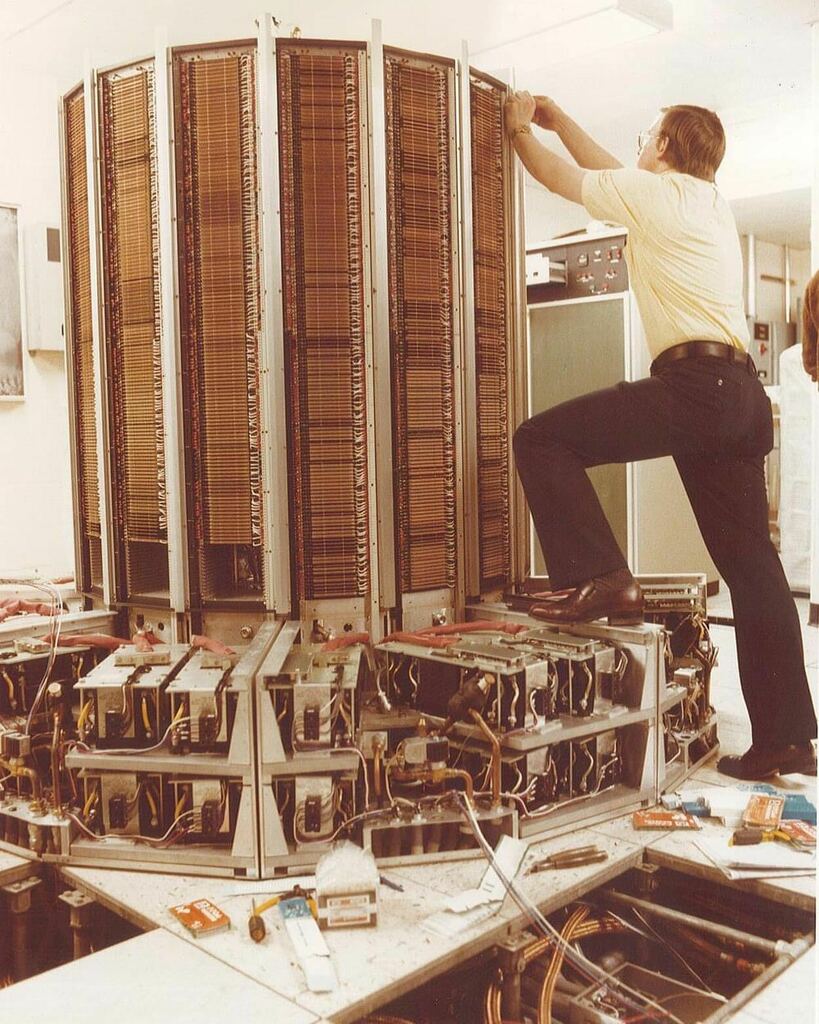In this faded 1970s photograph, a man is intensely focused on working on an intricate piece of technological equipment, possibly an early computer system. Dressed in a white short-sleeve shirt, black pants with a black belt, and brown leather shoes, he stands with his left foot elevated on part of the machinery. His thick-framed glasses and side profile suggest his concentration as he manipulates a vertical, cylindrical structure made up of multiple electronic components and layers that resemble routers or computing boxes, meticulously stacked and interconnected. The room around him is filled with additional boxes, cables, and computing devices that further anchor the scene in the 1970s era.